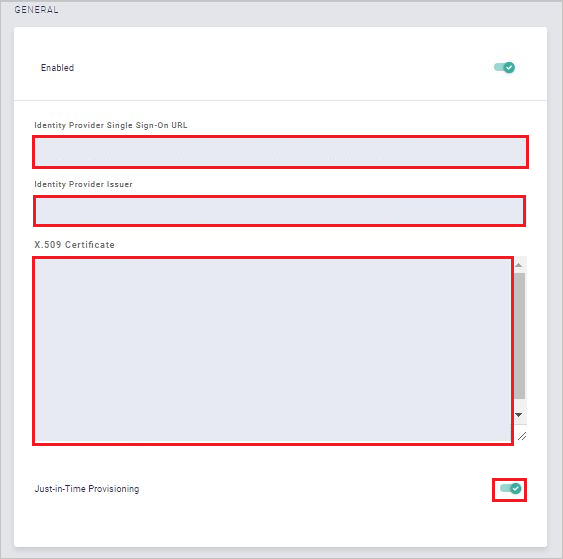The image features a vertical rectangular interface with a layered design. The outer background is a light bluish-gray, labeled "General" in gray text at the top left corner. Overlaying this background is a centrally placed white box.

At the top left of the white box, the word "Enabled" is displayed in bold black text. To the right of this text, there is an "on" button illuminated in bright blue, indicating an active state.

A thin gray line stretches across the top segment of this white box, dividing it from the content below. Directly beneath this line, there are three horizontal boxes, each with a light blue background framed by a bright red outline. The first two are narrow horizontal boxes. The top box is labeled "Identity Provider Single Sign-On URL" in black text. Directly below it, the second box carries the label "Identity Provider Issuer."

The third box is larger and also horizontal, identified by the label "X.509 Certificate" in black text. At the lower left corner of the white box, beneath the X.509 Certificate box, the phrase "Just-In-Time Provisioning" is printed in black text. Adjacent to it on the right, there's another "on" button set to active, lit up in bright blue and framed by a red outline.